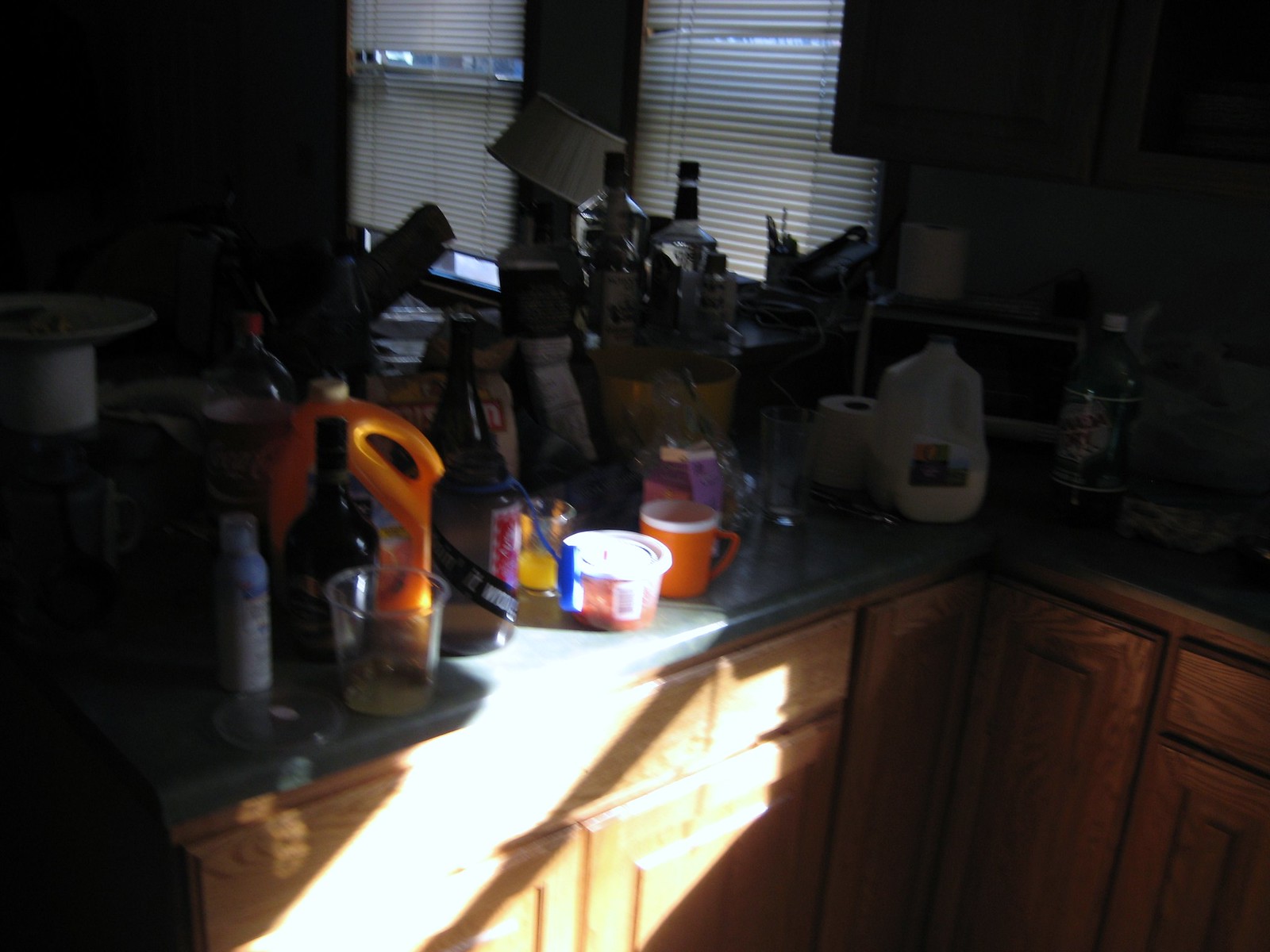The photograph captures a dimly lit kitchen at dawn, where the rising sun's angled rays illuminate select portions of the cabinetry and countertop. A small section of the counter is bathed in morning light, highlighting a plastic bowl with a lid, complete with a barcode indicating it's a store-bought item. The cluttered countertop features various items, including an assortment of glasses, a plastic mug, a less-than-half-full gallon carton of milk, and a two-liter soda bottle. A roll of toilet paper is inexplicably placed among the kitchen items. A yellow container, likely holding dishwasher soap despite the absence of a visible dishwasher, stands out. A glass Pyrex measuring cup is also present, alongside a wine bottle and several empty liquor bottles towards the back. The countertop is black, creating a striking contrast with the light brown wooden cabinets.